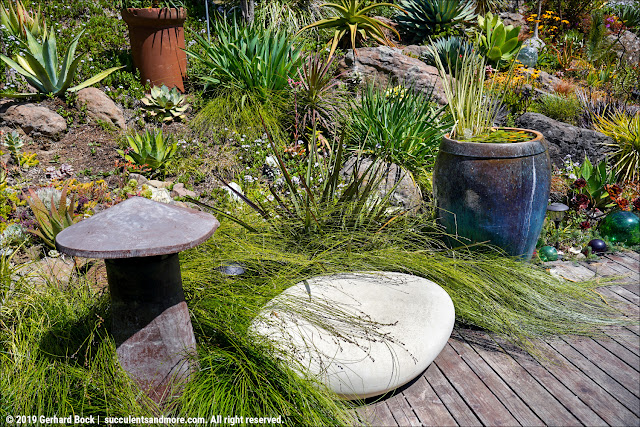This photograph captures an overgrown and natural-looking tropical garden, likely situated in a dry or desert climate. Central to the image is a large, smooth, white rock set against a landscape filled with various succulents, cacti, aloe, and spiky grasses. To the left of the rock is an intriguing mushroom-like sculpture, made of iron or wood, adding a quirky touch to the scene. To the right is a prominent blue vase filled with water, lily pads, and possibly some green shoots emerging from its surface. The lower right-hand corner features plank flooring, suggesting a wooden patio or deck area. In the background, additional interest is added by a rust-colored terracotta pot containing yet more plants. Scattered throughout the garden are vibrant splashes of color from flowers in yellow, orange, and purple hues. The bottom left-hand corner of the photograph contains white text reading "2019 Gerhard Bach, succulents and more.com, all rights reserved," confirming the image’s source and date.